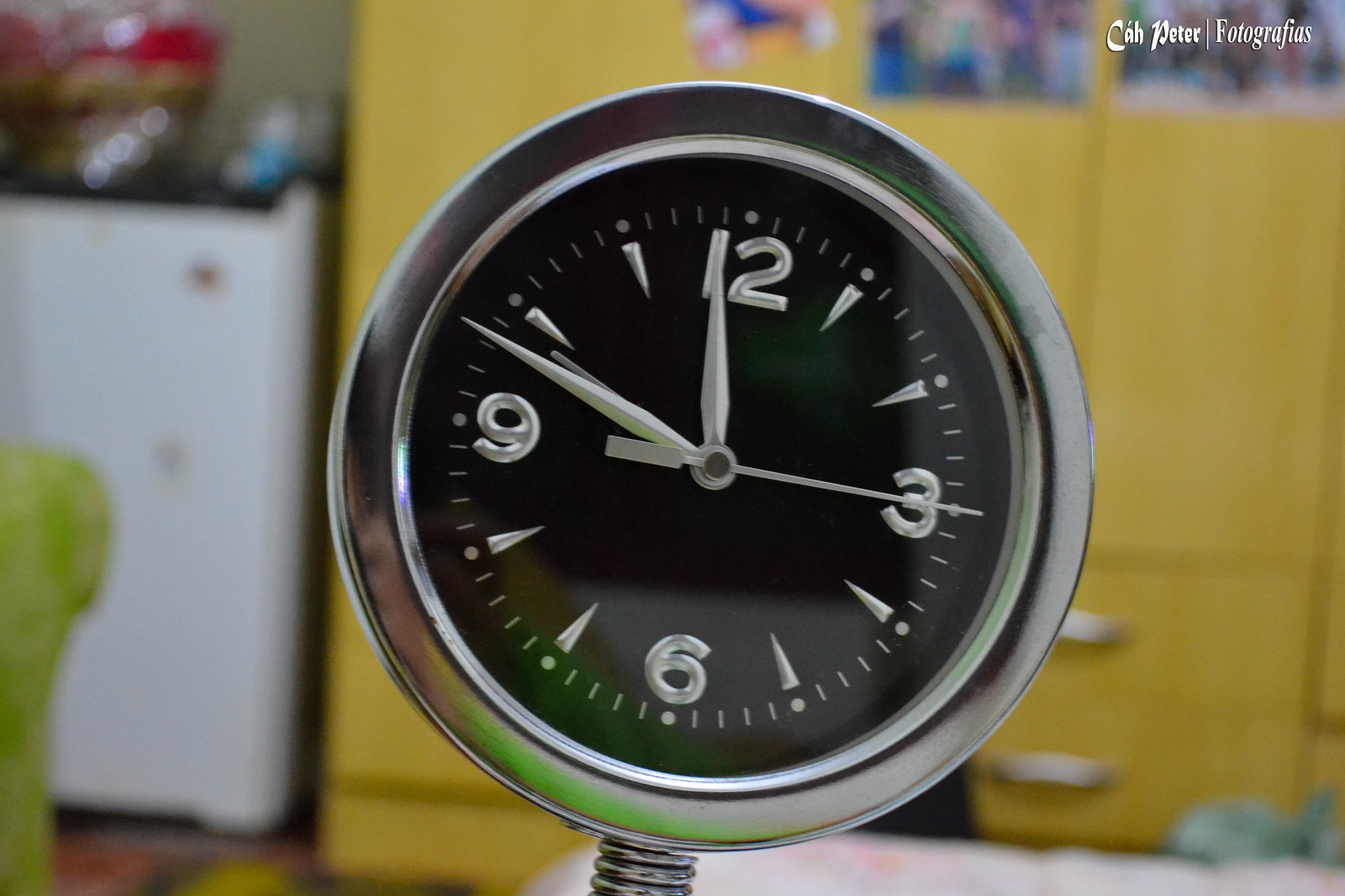This photograph captures a small clock, approximately three inches in diameter, mounted on a surface. The clock features a silver ring around its perimeter and a black face displaying the current time, 11:48. Extending downward from the bottom of the clock is a silver screw-like component. The background consists of a yellow cabinet and a white cabinet, each adorned with various indistinct items that are blurred in the image.